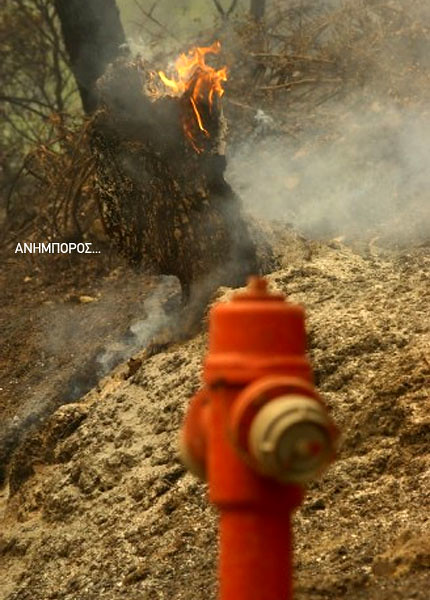The image captures an intense yet controlled scene of a forest fire, with a particular focus on a charred tree stump in the background and a partially blurry red valve with a golden attachment in the foreground. The valve, which could be mistaken for a fire hydrant, stands upright amidst a dimly lit setting engulfed in smoldering gray smoke. Surrounding the flaming stump, there's a noticeable pile of sawdust, suggesting the tree was deliberately cut down, possibly to initiate the burn and remove the stump. Among the ashy remains and dark brown, charred shrubbery, a moderate, orange-and-yellow flame is visible licking the base of the tree. The scene further includes some sparse greenery in the far background, indicating untouched parts of the forest. White uppercase letters in a small font—A-N-H-M-N-O-P-O-E—dot the upper left corner of the image, against a backdrop of chaos, adding a cryptic touch to this grim firefighting scenario.